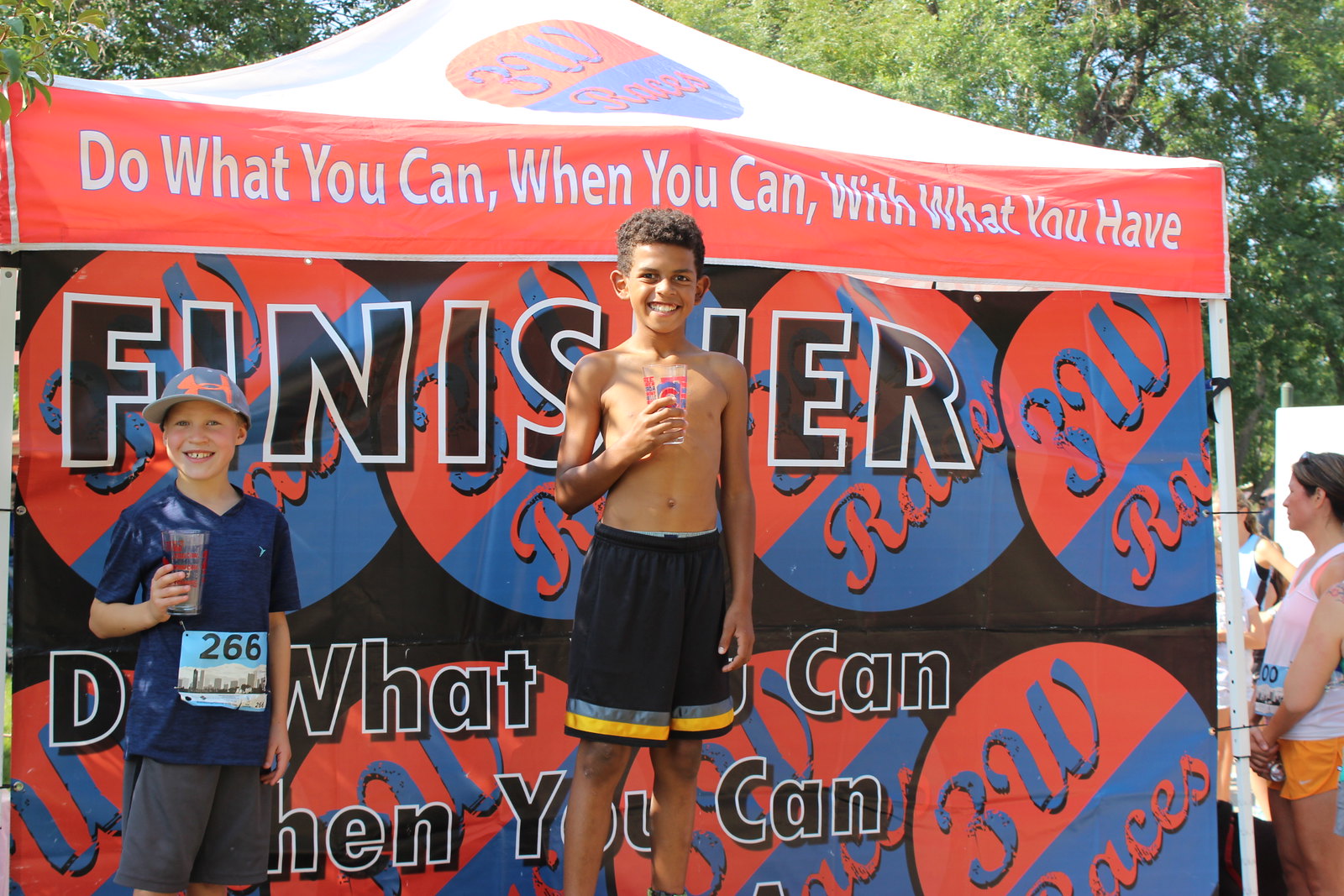In the outdoor setting of this lively event, two young boys stand in front of a colorful pavilion adorned with the inspiring slogan, "Do what you can, when you can, with what you have." The pavilion features a mix of red, blue, black, and white colors. The boy in the middle, with dark skin and short curly hair, smiles directly at the camera while holding a drink in a glass decorated with red and blue colors. He is dressed in black shorts with a gray and yellow stripe at the bottom and is shirtless. Next to him, another boy with lighter skin stands smiling, also facing the camera. He wears a light blue baseball hat with an orange "H" design, a blue collared short-sleeve shirt, and gray shorts. A paper pinned to his shirt displays the number "266" along with an illustration of what appears to be a cityscape against a blue sky. Both boys appear cheerful as they pose in front of the red and white pavilion tent, with tall trees visible in the background and a couple of people partially seen on the edge of the frame.